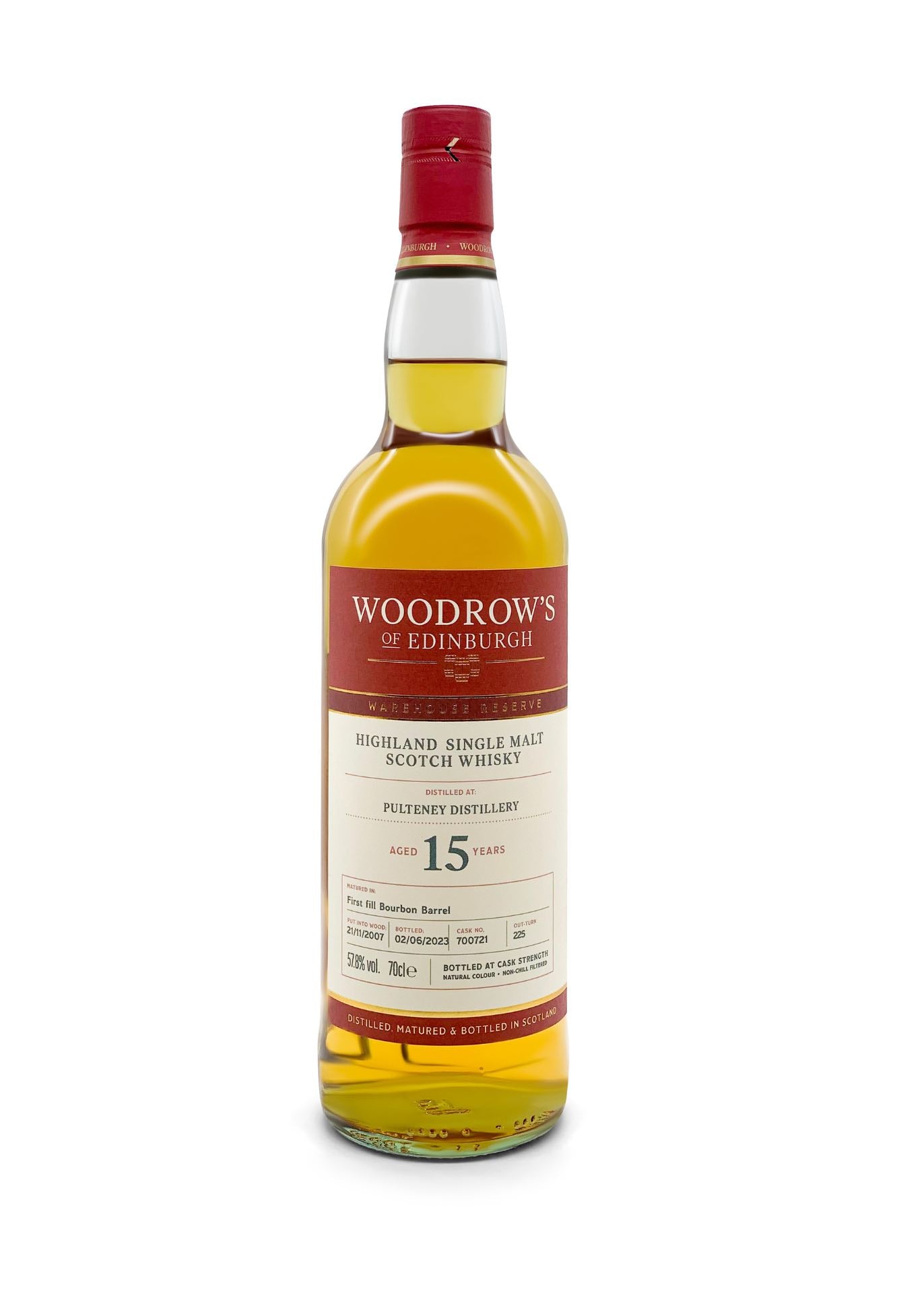This detailed color photograph shows a bottle of whiskey against a stark white background, focusing solely on the product. The whiskey within the glass bottle is a rich golden brown, filling the bottle up to the neck with a slight air gap at the top. The bottle is sealed with an ornate red and gold cap, featuring predominantly red wax with gold detailing and a band at the base.

The front of the bottle displays a large, intricate label divided into two sections. The top section of the label is red and reads "Woodrose of Edinburgh" in white letters, with a crest and the words "Warehouse Reserve" partially visible. The bottom section of the label is white and prominently showcases "Highland Single Malt Scotch Whiskey" in black text. Further down, the label indicates the whiskey is "distilled at the Pulteney distillery," aged for "15 years," with the number "15" featured boldly. Beneath this, smaller black text within a red grid provides additional details such as the volume, alcohol content, and distillation specifics, although these are hard to discern due to the fine print.